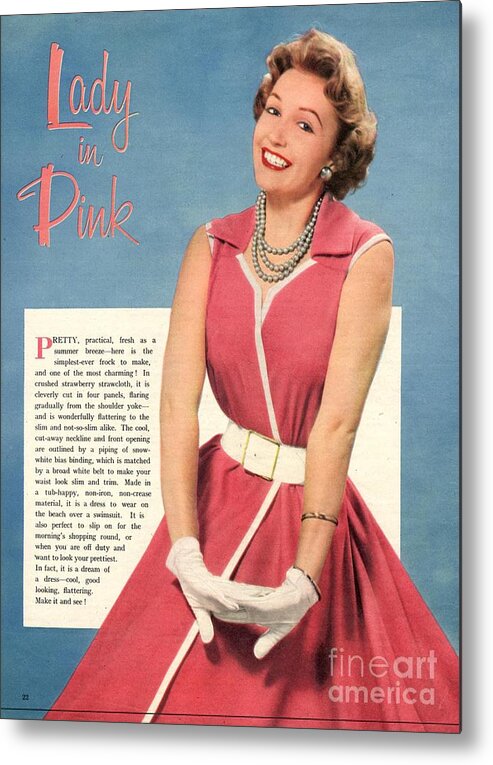The image is a vintage-themed poster with a copyright by Fine Art America, set against a blue background. Prominently featuring the title "Lady in Pink" in pink script in the upper left corner, it showcases a photograph that evokes the style of the 1960s or early 70s. The photograph centers on a younger woman with short brown or dirty blonde permed hair, sporting a vivid smile accentuated by red lipstick. She is adorned with a triple-layered pearl necklace and white gloves, her fingers interlocked in a poised manner.

The woman is elegantly dressed in a sleeveless pink frock that flares out past her knees in a flattering A-line fashion. The dress features a white border on the sleeves, a cool cutaway neckline detailed with snow-white bias binding, and a prominent thick white belt that accentuates her waist. Beside her, an article celebrates the garment's charm and practicality, describing it as a "Pretty Practical Fresh in the Summer Breeze" outfit made from a non-iron, non-crease material. The narrative highlights the frock as effortlessly wearable over a swimsuit at the beach or for casual morning errands, deeming it a dream dress that is cool, good-looking, and universally flattering.